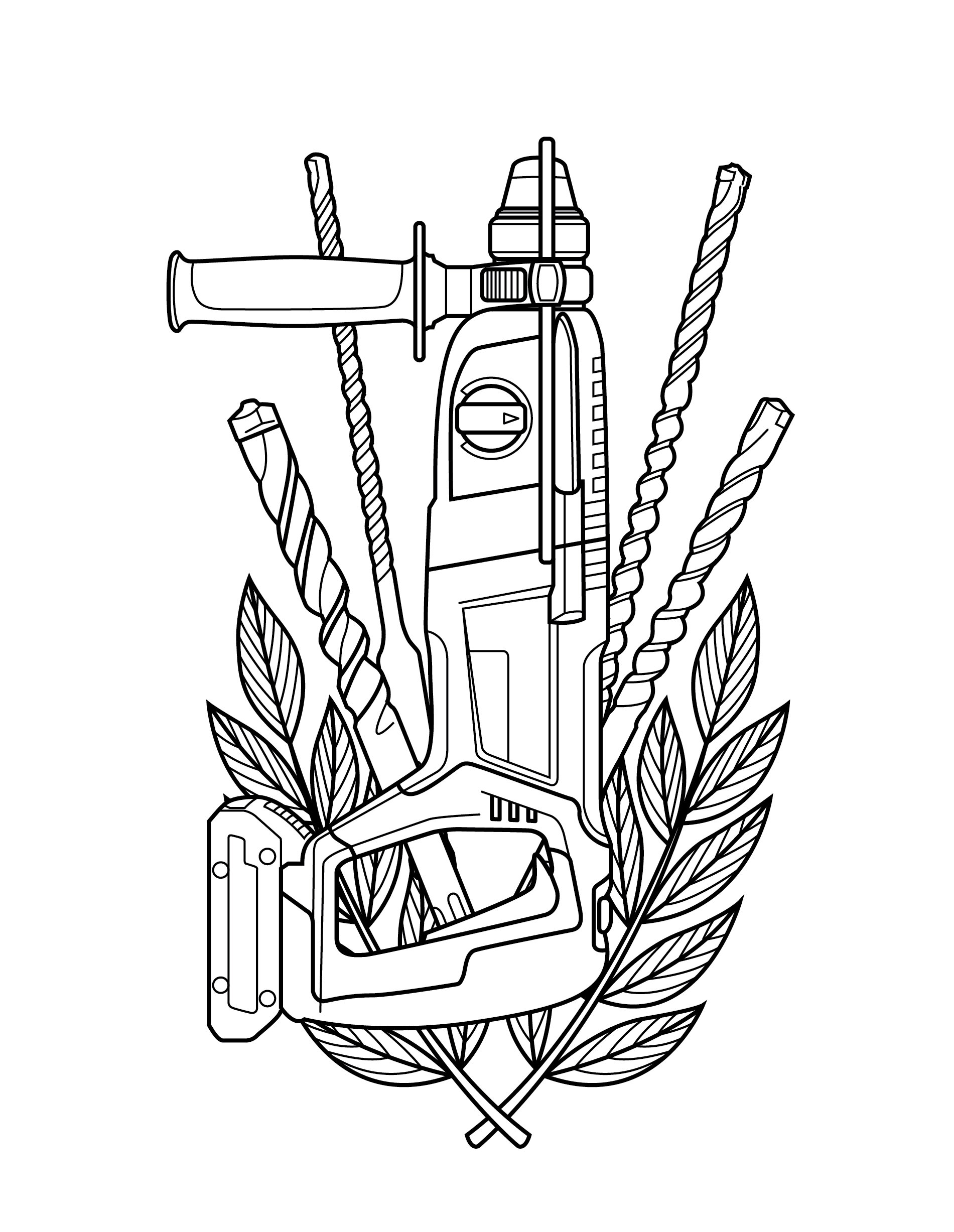In this black and white vector illustration, a detailed power tool, resembling a high-precision drill, is depicted facing vertically upward. The tool features a vertical foregrip attached to its barrel, with a small dial situated underneath the grip. At the rear, there is a compartment loaded into the bottom, suggesting the presence of a power source or additional tool attachment. The handle is equipped with a long trigger and a protective handguard, likely designed for safety and ergonomic use. Surrounding the tool are meticulously illustrated leaves, with two sets of nine leaves each, positioned at the base and extending upwards on stems. Additionally, there are four distinct types of drill bits, including a paddle bit, arrayed around the central tool. This intricate drawing, predominantly rendered in black ink with white accents, captures both the functional details and the artistic flair of the depicted objects.